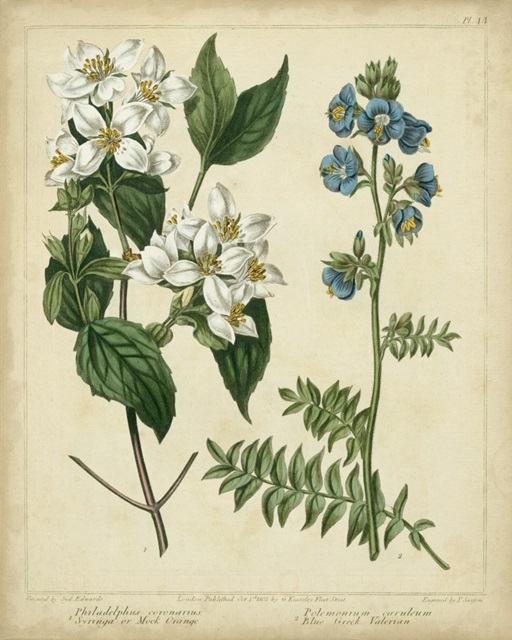This image features a vintage-style painting against a peach, almost beige, background, illustrating two distinct flowering plants. The left plant displays large, white flowers with four petals encircling numerous tiny yellow stamens at their centers, alongside sizable, broad green leaves. The right plant contrasts with smaller, delicate blue flowers and more numerous, closely-packed, arrow-shaped leaves, accompanied by several unbloomed buds. The painting has an overall aged appearance, emphasizing the vibrant green stems and foliage. The bottom of the image contains blurred writing, one word appearing to be "Valoran" and another, possibly "Corleum," though it is less clear.